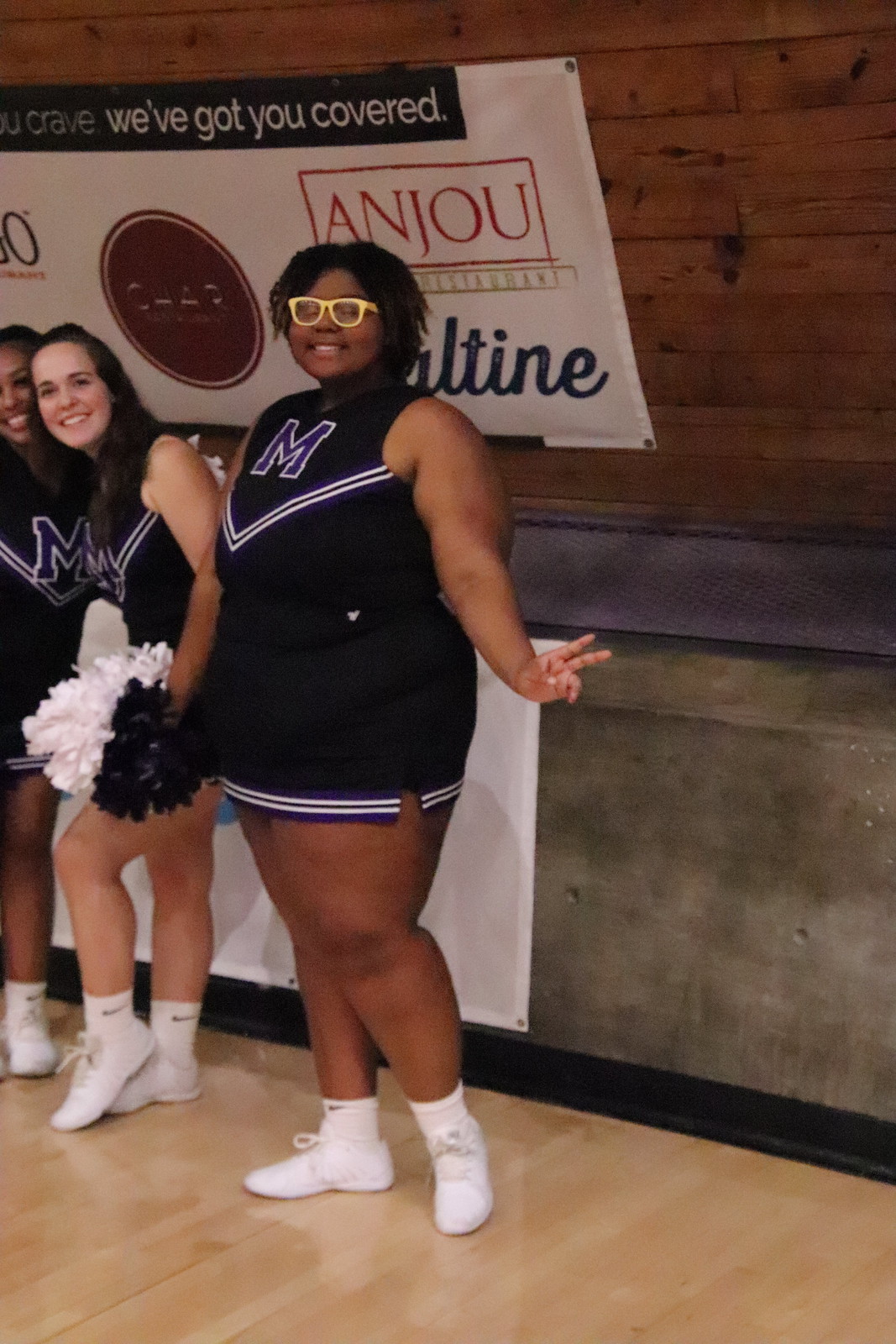In this candid color photograph, three female cheerleaders pose against the wall of what appears to be an indoor gymnasium. The central focus is on a plus-size, dark-skinned black cheerleader standing prominently at the far right. She is attired in a striking black cheerleading uniform accented with a purple "M" on her chest and white lines forming a V shape from armpit to armpit. Her skirt also features a white line around the hem. She completes her look with white ankle socks and white shoes. Her curly hair is parted down the middle, framing her face and partially covering her ears, while a pair of yellow-framed glasses adds a pop of color to her uniform. With a smile on her face, she extends her left hand to the right, flashing a peace sign, while her right hand rests naturally by her side. 

Flanking her are two other cheerleaders, partially visible at the edge of the photograph. To her immediate left is a thin white cheerleader leaning slightly to the left, and next to her is another black cheerleader, whose presence is just hinted at by the cut-off edge of the image. Both are dressed in identical black uniforms featuring the same white and purple accents, white socks, and white shoes. One of them holds blue and white pom-poms.

Behind the trio, a gray concrete wall serves as the backdrop. A white banner hangs prominently above them, emblazoned with the words "Crave. We've got you covered" on a black background, with a second section that has a white background displaying the word "ANJOU." This banner is mounted to a wooden wall, adding a touch of texture to the scene. The glossy wooden floor beneath them reflects the light, enhancing the indoor setting of this spirited moment.